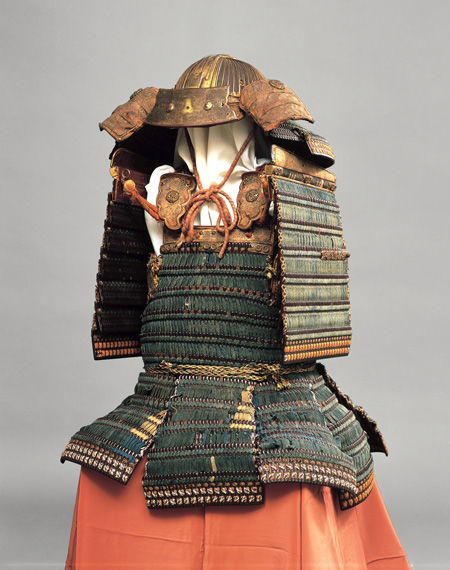This image showcases a historical samurai armor set displayed on a cloth-draped stand, presumed to be within a museum setting. The background of the image is gray, which contrasts with the vibrant orange tablecloth draped over the table where the armor is placed. The armor itself is a striking turquoise color, patinaed with age and adorned with intricate beaded designs and metal accents. The torso is protected by a chest plate, and shoulder straps extend to articulated shoulder panels. Below the chest plate, additional panels form a skirt-like arrangement around the waist, intended to drape over the tops of the legs. The long metal arm pieces and the bronze or brass helmet, complete with an orange cord for securing under the chin, add to the detailed craftsmanship of the piece. Despite minor damage indicative of its age, the armor remains remarkably well-preserved.